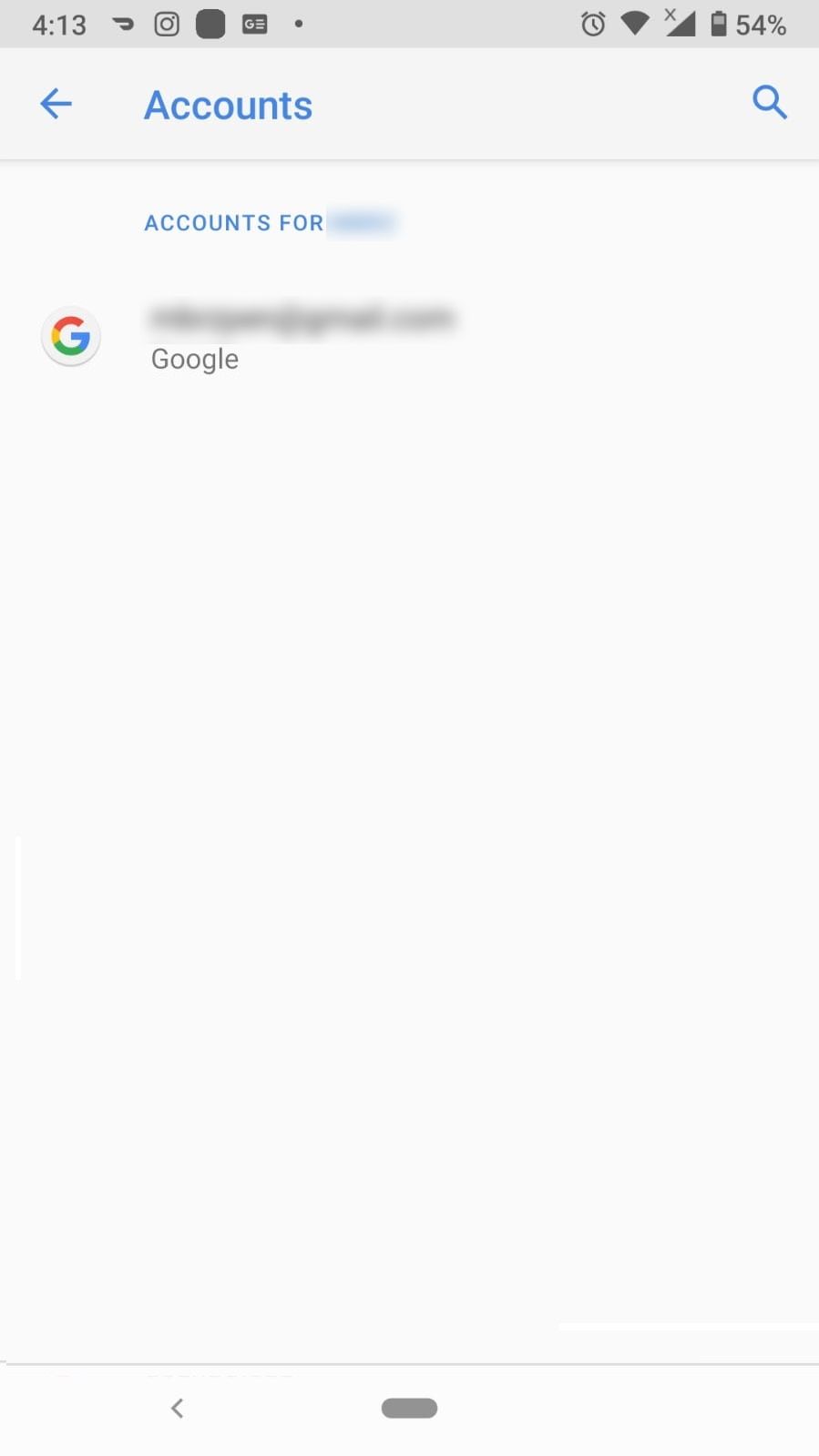This image depicts a smartphone screen with a predominantly white interface. At the very top, there is a light gray banner containing various icons and text. From left to right, the banner displays a time reading of "4:13," followed by an icon. Continuing right, there is a camera icon next to a dark gray square. Adjacent to this is a small rectangle containing the letter "G," followed by a small dot. On the far right side of the banner are a clock icon, a signal strength icon with a full set of bars topped by an "X," and a half-full battery icon indicating 54% charge.

Directly beneath this banner is the word "accounts" in blue, accompanied by a left-facing arrow and a blue magnifying glass icon. Below this line, the text "accounts for" appears, with the subsequent word blurred out in blue.

The left portion of the next segment features the Google icon, next to which are some blurred out words, with the word "Google" legible right below them. This section is followed by a substantial blank white space. Finally, at the very bottom of the page lies a gray oval.